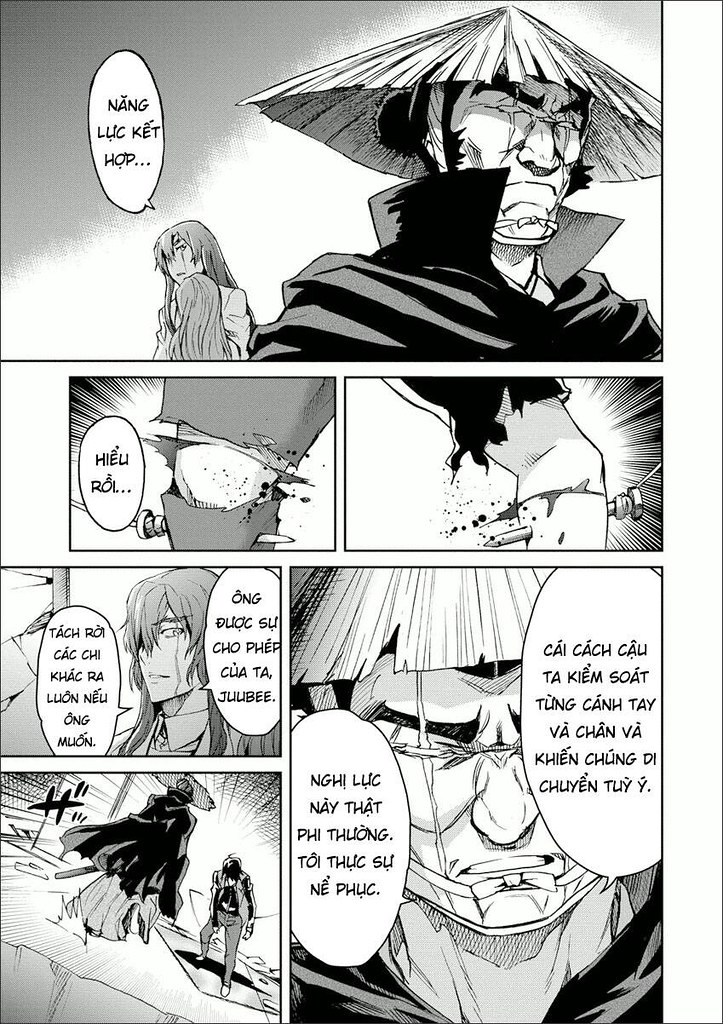This black and white image from a manga, likely Japanese in style but containing dialogue in a language that could be Vietnamese or Cambodian, features six intricate frames. The top frame highlights a man wearing a traditional Vietnamese-style conical hat and a black coat, facing the camera. His face is partially obscured due to cowering, and behind him stands a smaller woman with long hair, looking backwards with an expression of fear. She has a dialogue bubble in an unreadable foreign language.

The lower frames present disturbing details, including human knees being injured, penetrated by screws, conveying a scene of great distress. On the left side, one frame shows an image of the woman, and below that, there are two more figures. On the right side, the man in the conical hat reappears, this time facing forward, surrounded by text bubbles written in the same foreign language. The overall composition emphasizes tension and interaction between the man and the woman, with the monochrome palette adding to its intense, dramatic narrative.